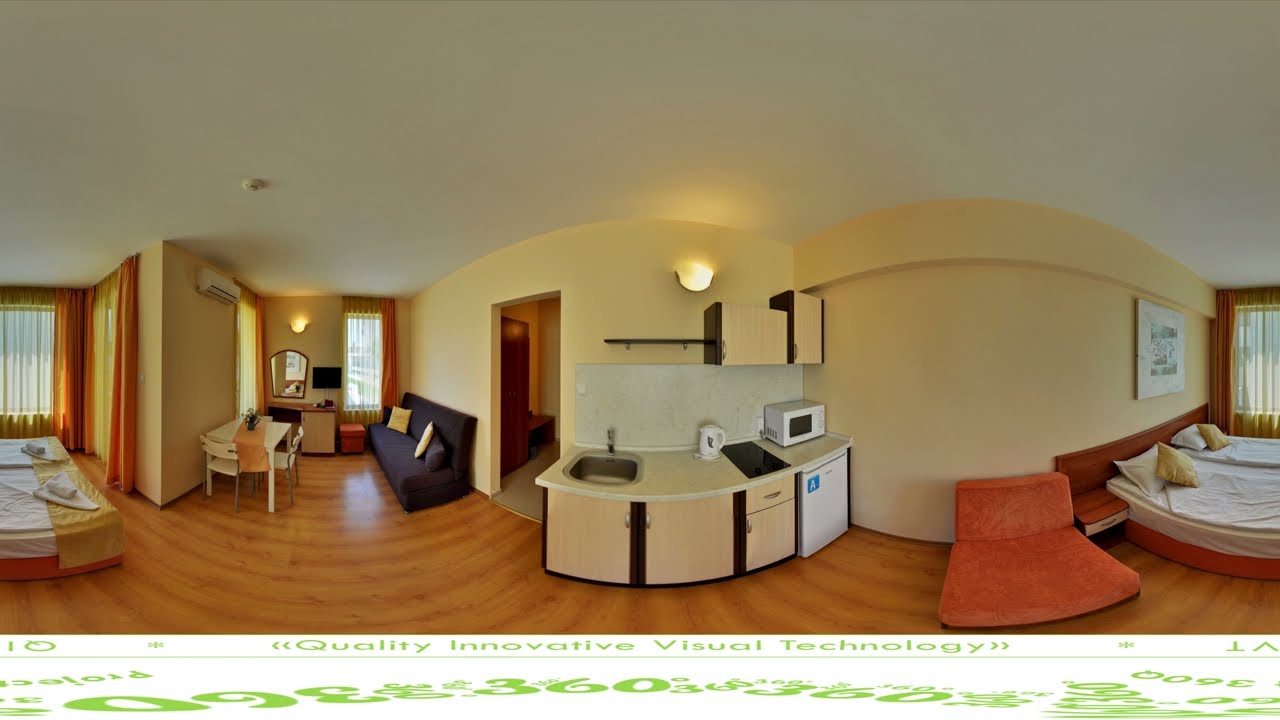This image showcases a vibrant outdoor pool area under a clear blue sky with the sun shining brightly in the top-left corner. The swimming pool, situated on the left side of the image, has clear green water, providing a refreshing contrast to the surroundings. The pool area is surrounded by a variety of white lawn chairs; more are visible on the right side, with some aligned neatly along the left. Blue umbrellas are interspersed among the chairs, providing shade. The ground around the pool is covered with tiles. In the background, there are several buildings, which appear to be part of a hotel or an apartment complex. Most buildings are three stories high, although there's mention of a two-story, peach-colored building in the middle. The entire scene seems to be shot with a VR lens, giving it a slightly distorted view, possibly implying a 360-degree capture. At the bottom of the image, there's green-on-white text that reads "Quality Innovative Visual Technology."